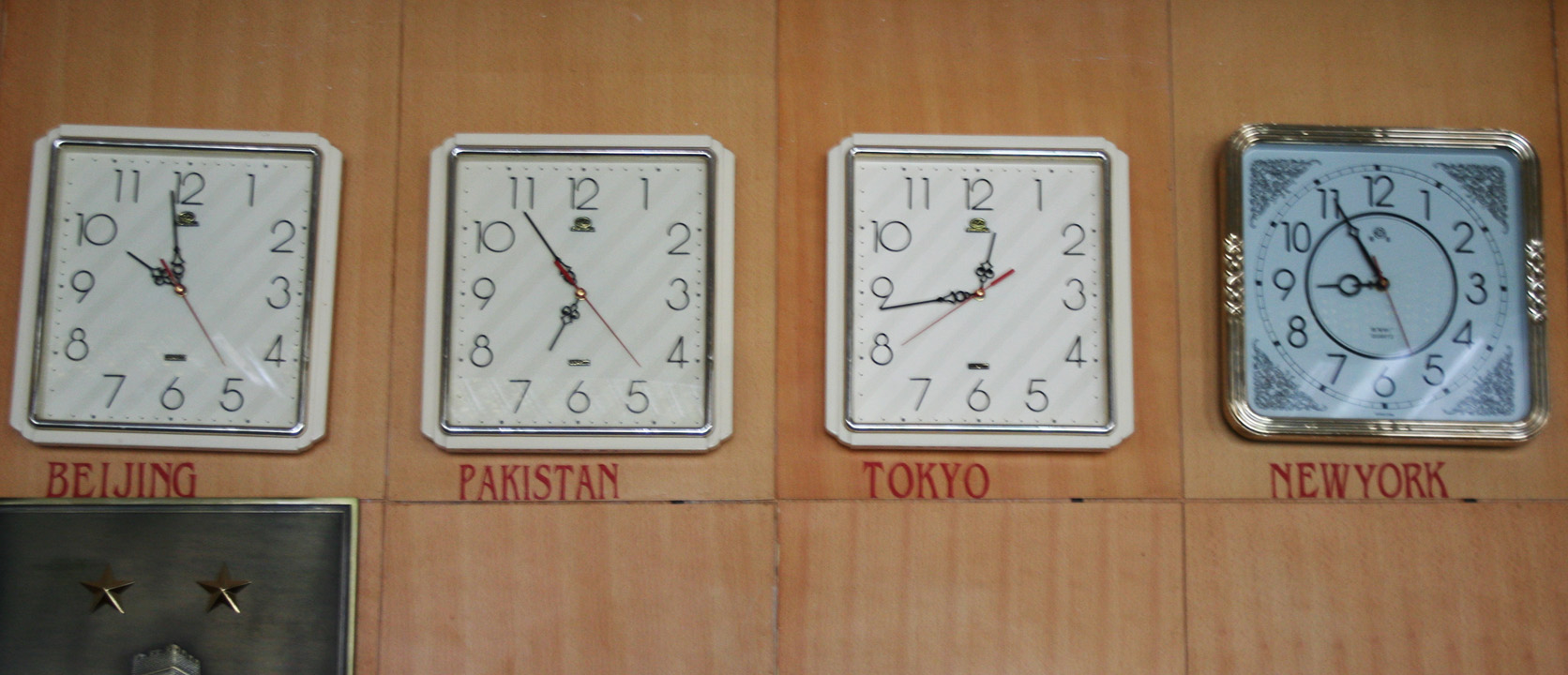This color photograph showcases four square, analog clocks mounted on a beige, wallpapered wall. Each clock displays standard numerical digits rather than Roman numerals. They all feature black minute and hour hands, alongside a red sweep second hand. Beneath each clock, the names of major cities are labeled in red: from left to right, Beijing, Islamabad, Tokyo, and New York. The times shown are precisely synchronized to each location: in Beijing, it is one minute to ten; in Islamabad, it is five minutes to seven; in Tokyo, it is. Finally, New York displays a time of five minutes to nine.